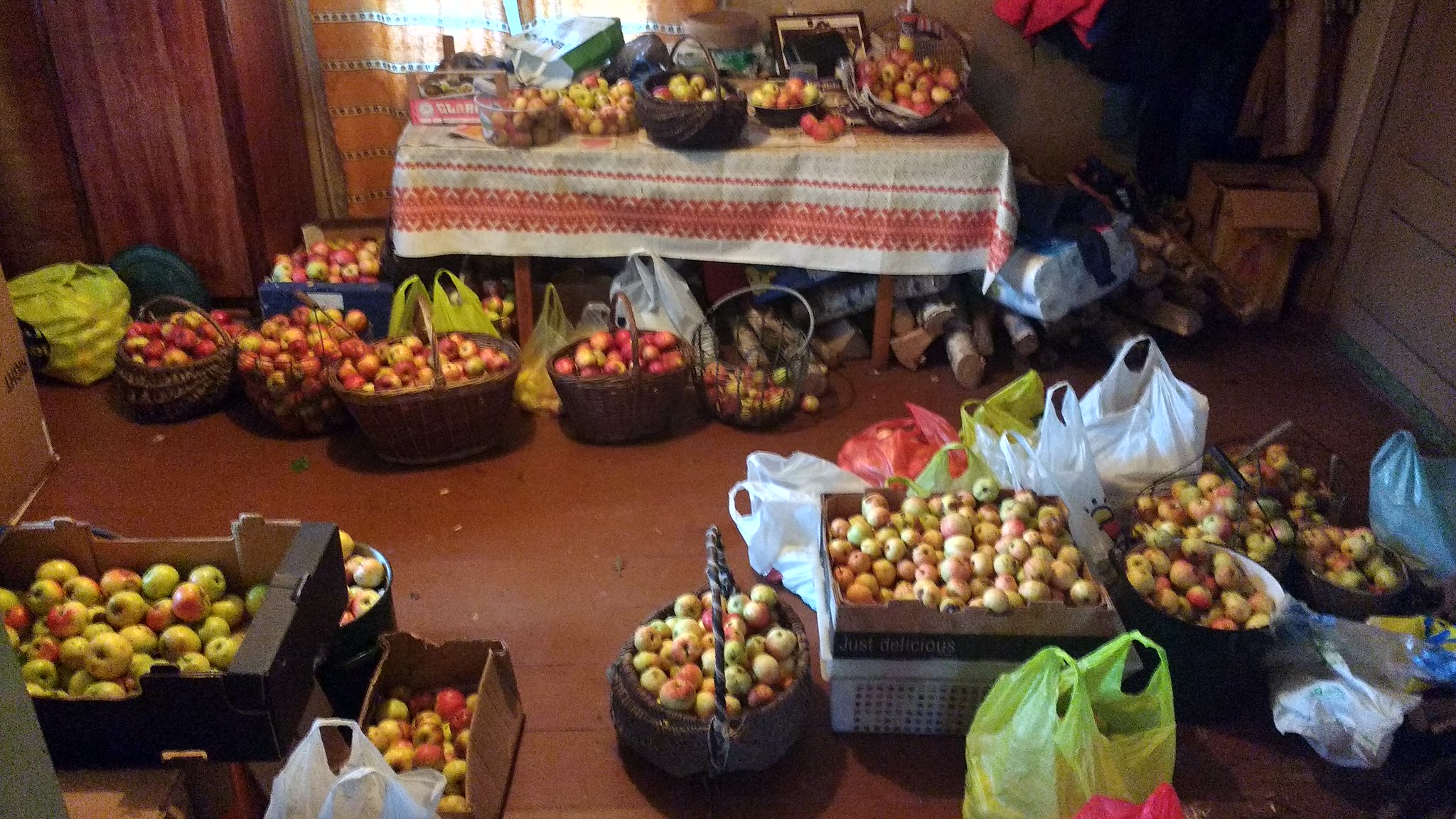The image captures an indoor scene dominated by an abundance of apples. The room is partially visible and angled slightly downward, providing a comprehensive view of the apple-filled space. In the foreground, a variety of containers overflow with apples, including plastic grocery bags, waxy cardboard produce boxes, and large woven wooden baskets. The apples themselves are small, displaying a mix of red, green, and yellow shades, reminiscent of Fuji apples.

Towards the back of the room, a table stretches across the scene, covered with a colorful blanket that features red and white patterns, possibly of Navajo design. This table is laden with baskets, bowls, and bags, all brimming with apples. Behind the table, light filters through sheer curtains on a window, adding a soft glow to the setting. The table also holds a photograph, adding a personal touch to the scene.

To the right of the table lies an unopened case of toilet paper, positioned on its side atop a heap of miscellaneous debris. Beneath the table, wooden logs, likely birchwood firewood, are casually placed, adding to the rustic ambiance. In the top right corner of the image, a box is visible near a closed brown door.

The entire room seems to be meticulously organized to showcase the apples, with a clear walkway through the strewn containers, suggesting a purposeful and inviting arrangement for easy access. The rich variety of apple containers and the room's functional yet cozy décor hint at a setting that might be part of a fruit stand, an apple orchard’s indoor shop, or a bulk-buying area for fresh produce.